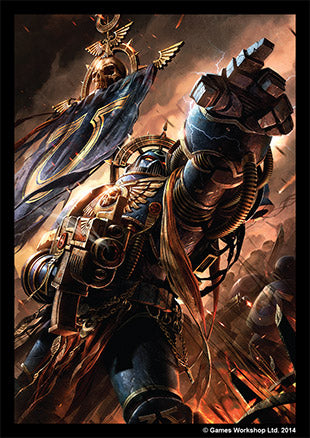This illustration is an intricate, detailed, and steampunk-inspired graphic artwork, potentially derived from a collectible card or gaming poster. The image, framed by a black border and presented in portrait orientation, features an armored figure dominating the scene. This imposing character, predominantly clad in metallic blue armor with copper accents, is adorned with an array of gizmos, tubes, and weapon-like appendages. He extends a formidable, armored finger into the distance. The coppery-gold metallic background, resembling either a sky or flames, imbues the scene with a fiery essence.

In the background, a flagpole rises behind the main figure, topped with a gold skull and flanked by vaguely Nazi-like eagles. Beneath the skull extends a blue banner, while another element, a metal skull with outstretched arms and a black flag or sail adorned with a gold symbol, appears in the top left corner. Shadows that may suggest an army or followers loom faintly behind the armored figure, hinting at an impending march or battle. In the bottom right corner, the image is branded with the copyright "Games Workshop LTD, 2014," indicating its origin. The dark, orangey, and coppery hues of the background contribute to the overall dystopian and mechanical atmosphere.